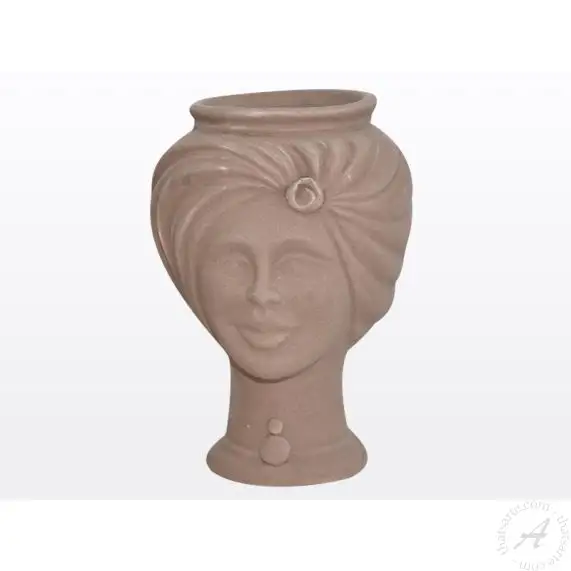This detailed picture showcases a unique and elegant vase designed in the shape of a woman's head. The piece, rendered in a rich chocolate brown hue, features intricate details: the woman's face is visible with slightly pursed lips forming a subtle smile, a defined nose, and eyes that appear to be closed in a serene expression. The vase depicts her head adorned with a turban-like scarf that covers most of her hair, save for a distinct round curl positioned above her forehead just below the vase's opening. A noticeable feature includes the woman's neck adorned with a necklace, highlighted by a round medallion at the center. The vase stands on a short base that begins at the woman’s mouth or cheekbones. With its combination of detailed facial features and decorative elements, including the turban and necklace, this vase would make an exquisite addition to any collection, blending artistry with functionality.